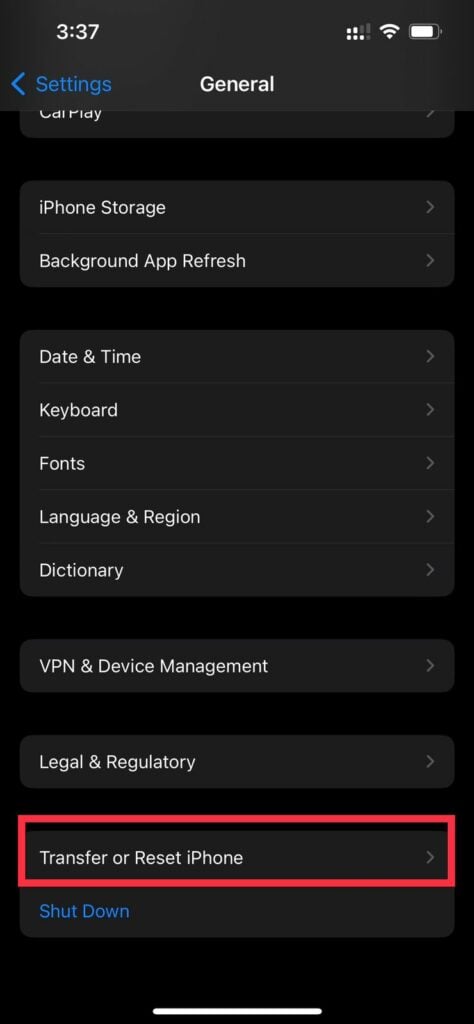The screenshot showcases an iPhone settings menu with various options listed in white text on a black background. Key settings include Wi-Fi, battery, general, iPhone storage, background app refresh, date & time, keyboard fonts, language & region, dictionary, VPN & device management, legal & regulatory, and Transfer or Reset iPhone. There is a distinct red box highlighting the 'Shut Down' option, which is presented in blue letters. A white bar is visible at the bottom of the screen, potentially indicating open apps or navigation options.